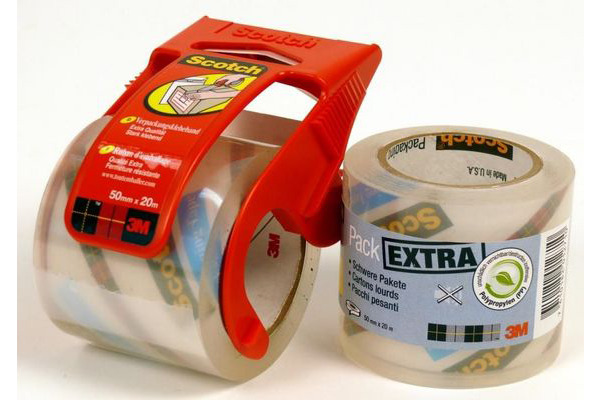In this image, there are two rolls of clear Scotch packing tape, manufactured by 3M, arranged side-by-side against a clear background. On the left, a roll is housed in a red dispenser adorned with a red label featuring the word "Scotch" at the top. Below this, there is an illustration depicting the application of the tape on a package, followed by a description of the tape’s dimensions (50 mm by 20 m) and the 3M logo. To the right, there is an extra roll of tape with a blue label that prominently displays the words "Pack Extra" in white and black letters. Accompanying this text is an image of a leaf and the word "polypropylene." Additional text and a barcode are also visible on the label. Both tapes are clear, making them suitable for packing and mailing packages efficiently.